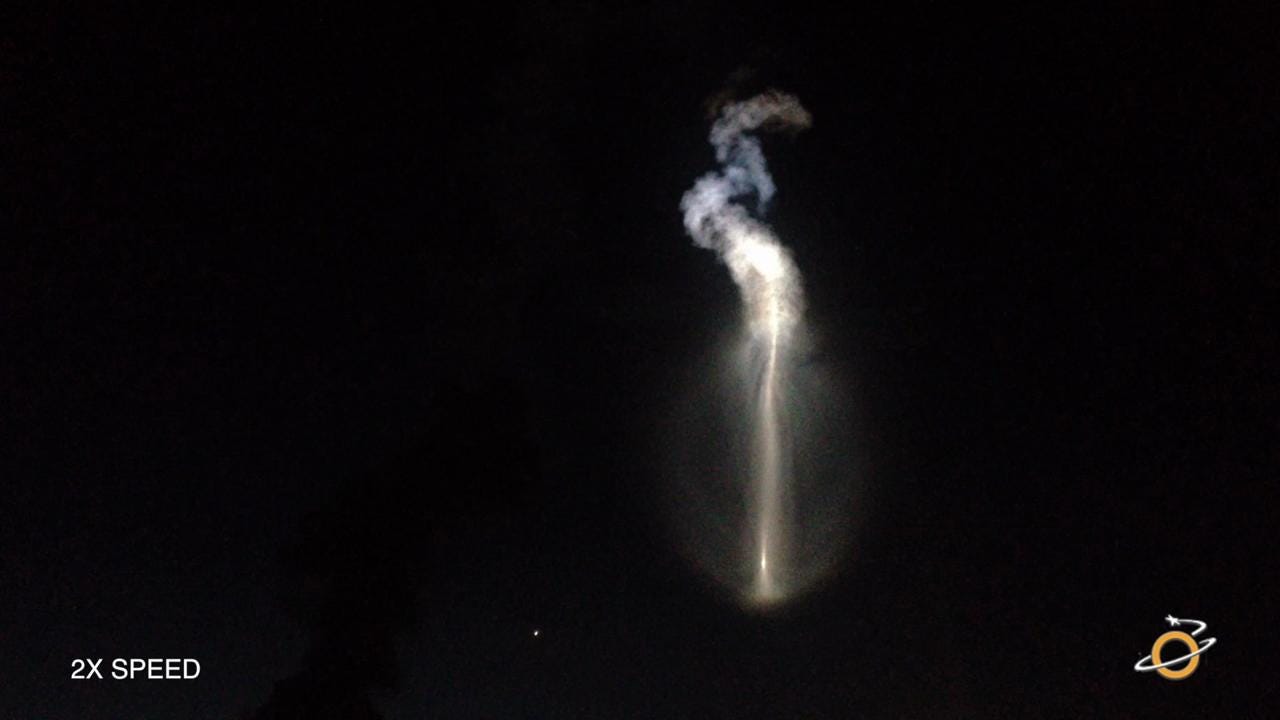The image is a colored photograph taken outdoors during the night, with a pitch-black background. Dominating the center of the picture is a striking display of white light, starting from an oval shape at the bottom. This light forms a pillar that shoots upwards and slightly curves, resembling a tube. The light is brightest at the bottom, creating a vivid focal point that gradually fades as it ascends. At the top, this pillar of light culminates in a shape reminiscent of a mushroom, where the light becomes more dispersed and grayish, nearly turning black. Along the lower left corner of the image, the text "2X SPEED" is clearly visible in white capital letters. On the lower right, there is a distinctive logo consisting of an orange circle encircled by a white ring, similar to a planet with an orbiting star. This photograph likely captures something moving through space at high speed, with a lingering white cloud trailing behind the object.